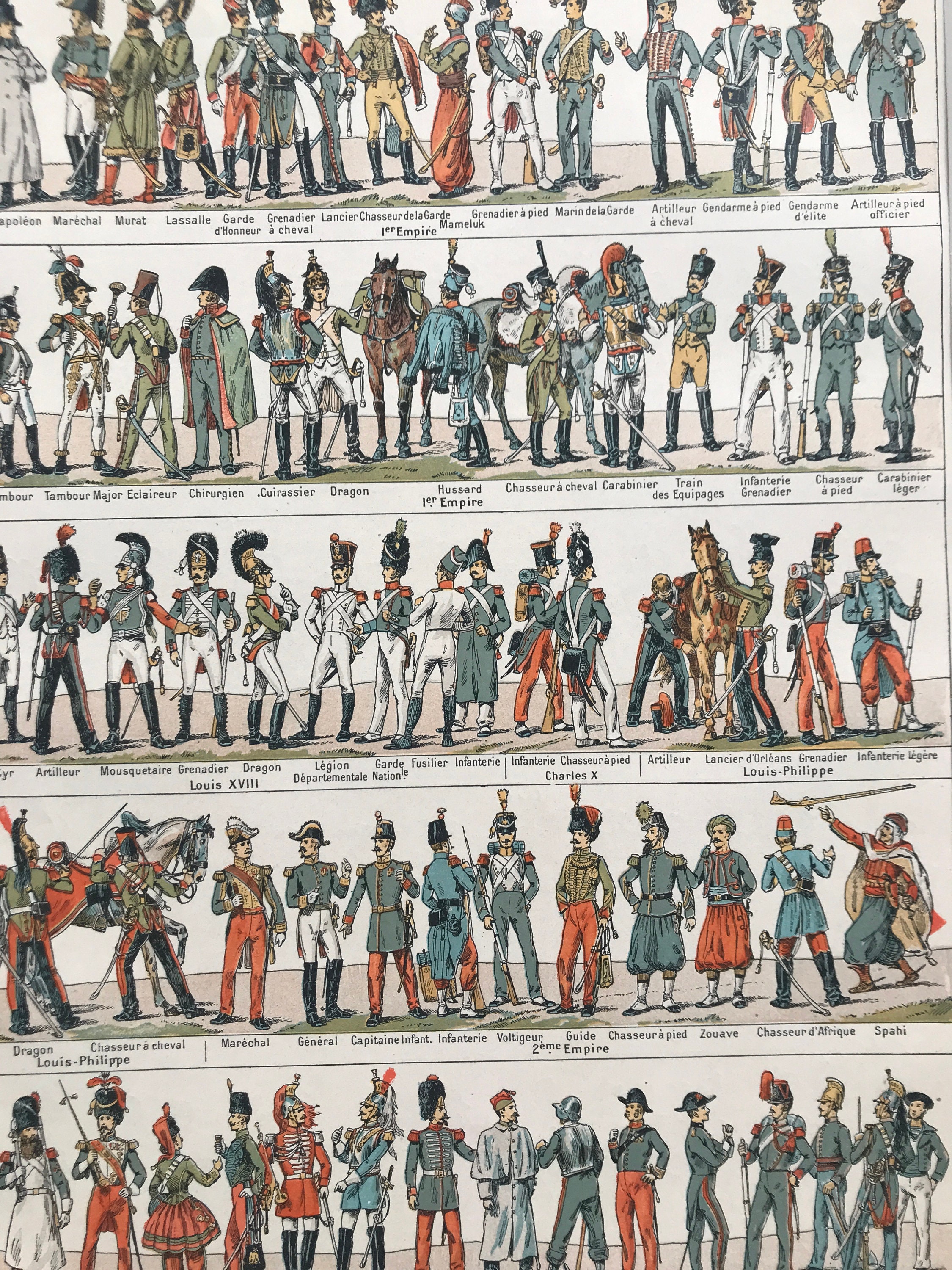This vintage illustration, likely a page from a French military history book, showcases approximately 75 to 100 soldiers arranged in five rows of 15 to 20 men each, spanning a period of 100 to 200 years. Each soldier is depicted in a distinct, meticulously detailed uniform, highlighting the rich diversity in military attire from various eras and units. The soldiers stand proudly in an array of colorful and muted hues, predominantly in blues and golds, with a middle row featuring individuals in uniquely white uniforms. Beneath each figure, there are small, presumably descriptive French captions, though the text is too fine to discern specific details. Among the soldiers, three horses and an assortment of weapons, including swords, guns, and bayonets, add to the intricate tableau, painting a vivid picture of historical military regalia.